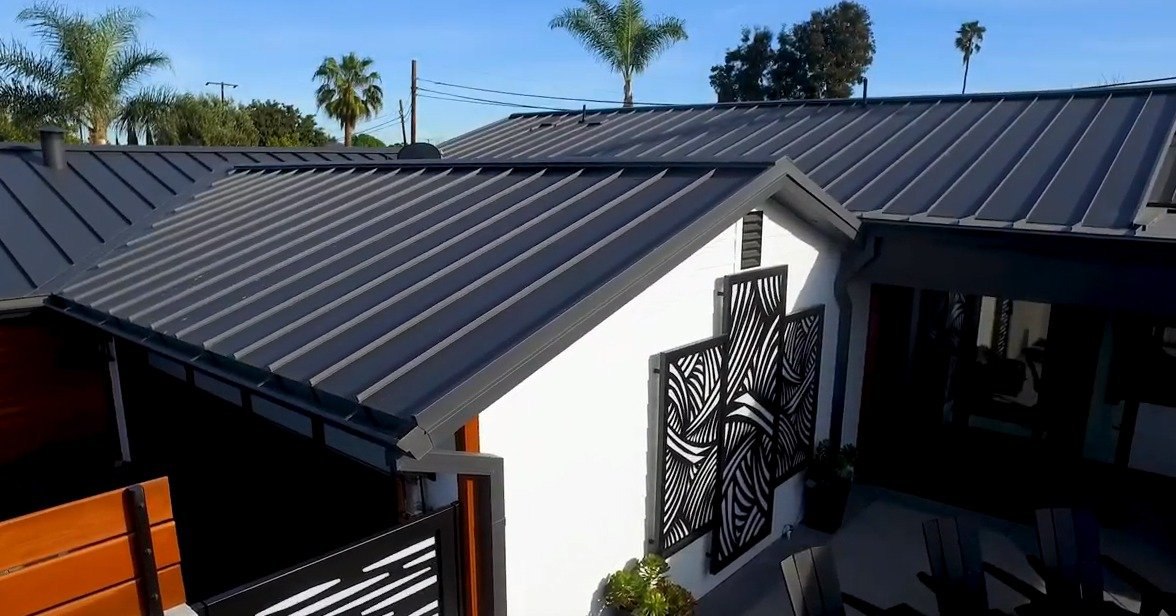The photograph captures a top-down view of a house taken on a bright summer day, showcasing a black-roofed, white-walled structure under a vivid blue sky. You can see part of the front or back of the house, where a significant feature is a striking black and white piece of art, possibly made of metal, shaped like a thick cross located on the exterior wall. Additionally, the house opens up to a patio furnished with black chairs, including Adirondack-style ones, and a small green bush. In the background, tropical palm trees and power lines are visible, enhancing the serene yet connected atmosphere. The gate in front is detailed with visible wood grain, and a little plant sits nearby, adding a touch of natural greenery to the scene.